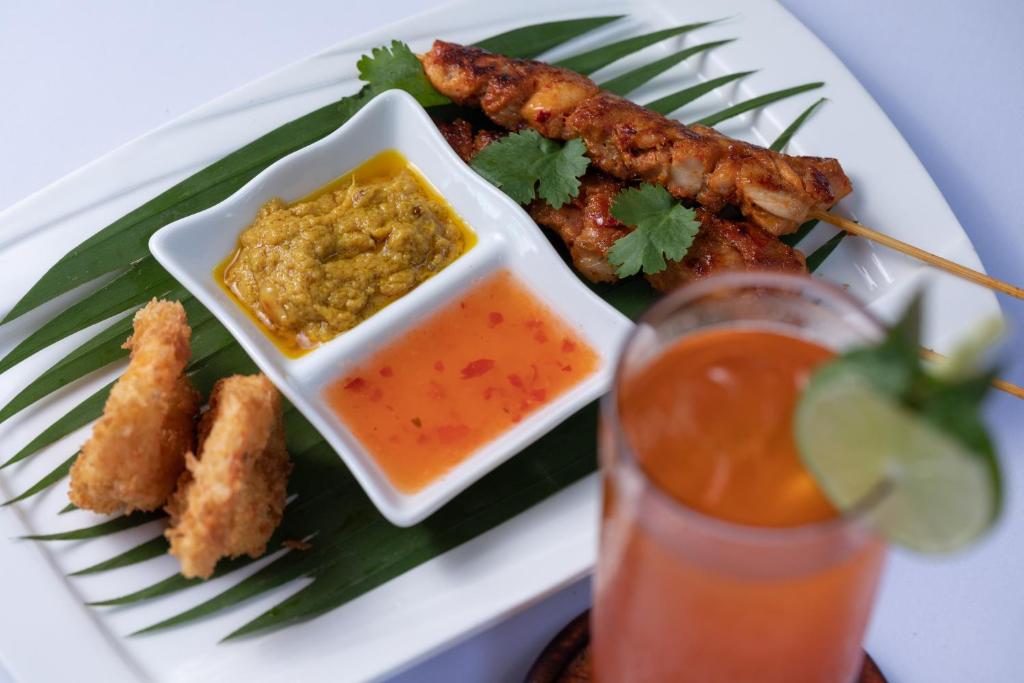The image captures a vibrant restaurant offering featuring a meticulously arranged satay dish as its focal point. The main dish is a large, white rectangular porcelain platter adorned with a decoratively fringed banana leaf. Resting on the banana leaf are two golden brown skewers of chicken satay, garnished with fresh cilantro leaves. In the center of the platter, there's a smaller rectangular divided dish containing two vibrant dipping sauces: the bottom section holds a sweet chili sauce flecked with red chilies, while the top section contains a thick, yellow curry sauce with an oily sheen.

To the left of the satay, two appetizingly breaded and fried shrimp, recognizable by their panko-like crust, complete the arrangement. The platter is placed at a slight angle, adding a dynamic touch to the presentation.

In the foreground, slightly out of focus, sits a tall, ice-filled glass of iced tea or perhaps an orangish beverage, garnished with a lime wedge perched on the rim, bringing an additional refreshing element to the scene.